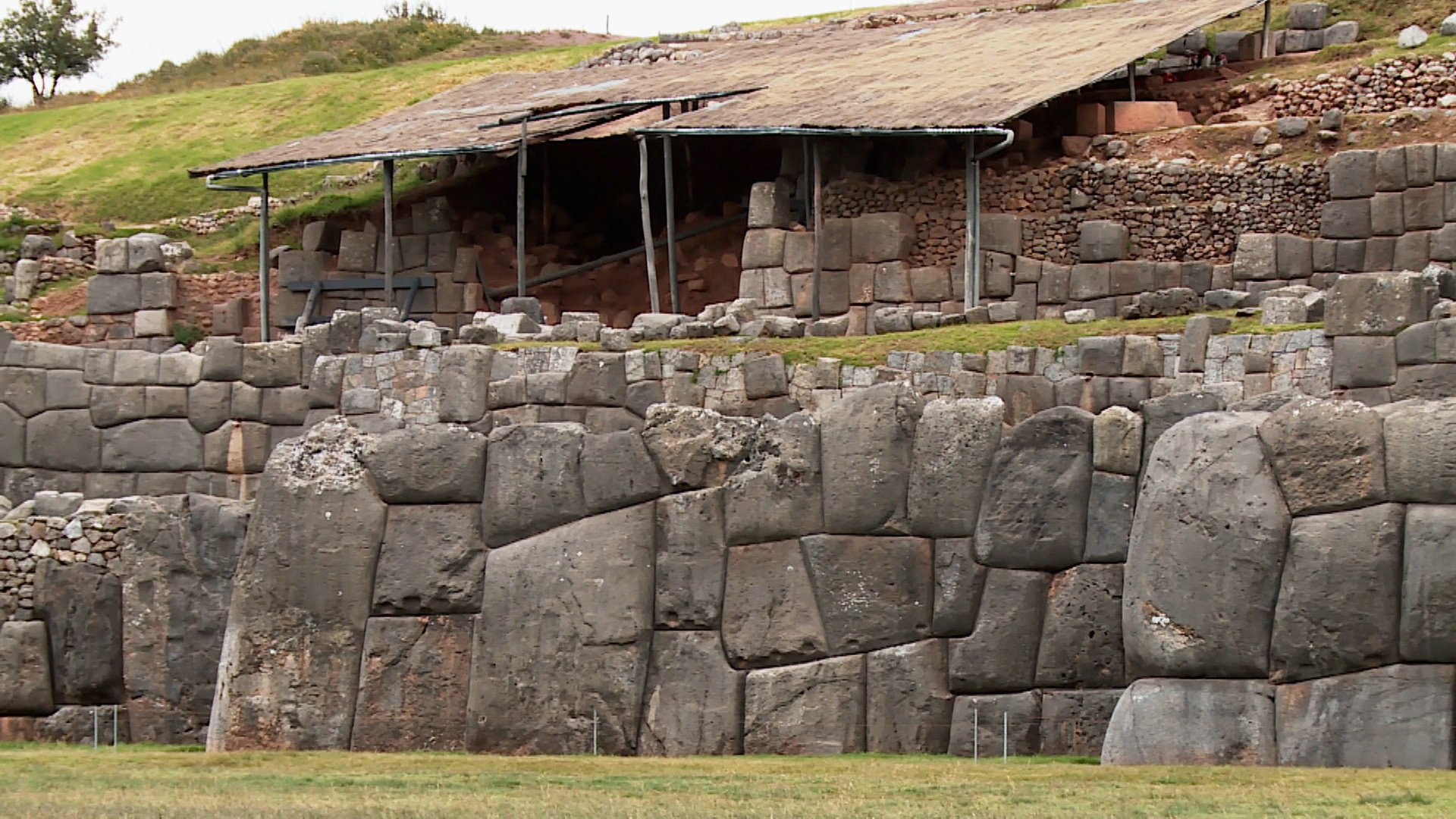This vibrant color photograph captures a terraced hillside adorned with meticulously crafted stone walls. The immediate foreground features a lawn with patches of yellow and green grass. Behind the lawn, a prominent stone wall constructed of perfectly cut and fitted stones spans horizontally. Ascending the hillside, a series of multi-tiered stone walls unfolds, each tier showcasing different sizes and shapes of stones. The stones range from large, rectangular blocks on the lower tiers to smaller, cube-like stones on the upper levels. 

Situated at the center of the image, amidst these stone tiers, is an intriguing shelter. It features an open stone wall construction with a sloped roof supported by wooden sticks. The roof, donned in weathered reddish and light brown hues, hints at a structure used for work or storage, as evidenced by the loose stones scattered beneath it. The shelter adds a touch of rustic charm to the landscape.

On the left side of the image, the terraced hillside continues to rise, leading up to a grassy area topped by a leafy green tree, positioned in the upper left corner. This combination of expertly constructed stone walls, the verdant hill, and the quaint shelter creates a harmonious blend of nature and human craftsmanship, resembling ancient but well-preserved ruins integrated seamlessly into the hillside.